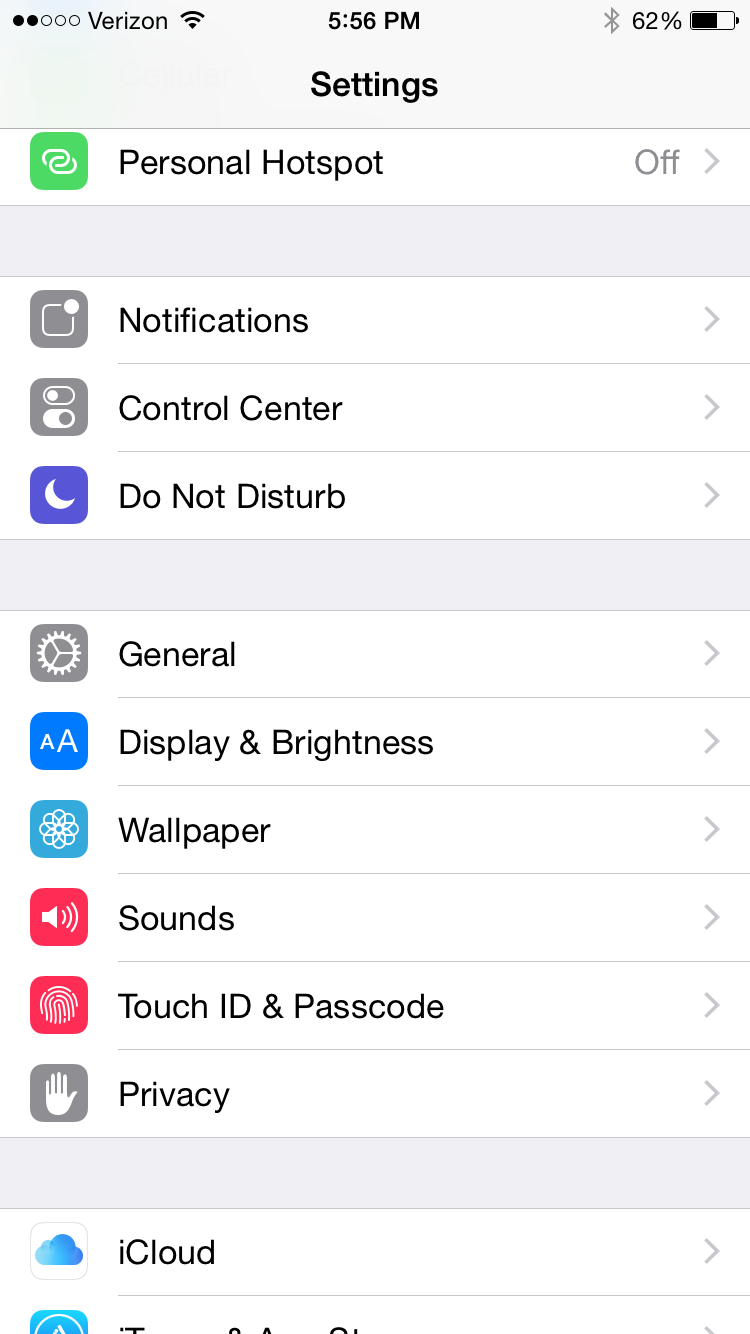This is a detailed screenshot of the settings page on a phone.

In the top left corner, there are two black circles side by side, followed by three white circles. Next to these symbols, "Verizon" is displayed in bold black text. Adjacent to the Verizon text is the Bluetooth symbol, characterized by a small circle intersected by two bars, followed by "5:56 PM." Moving right, another Bluetooth symbol is visible, accompanied by "62%" and a battery icon.

Directly below, the time "5:56 PM" is displayed again, followed by the word "Settings" in bold black letters. Underneath this, there is a green bar with the text "Personal Hotspot" to the left and "Off" to the right. 

Below this section, various boxes representing different settings options are listed:

1. A gray box labeled "Notifications."
2. Another gray box labeled "Control Center" next to a blue box featuring a white crescent moon symbol, which signifies "Do Not Disturb."
3. A gray box with a gear icon labeled "General."
4. A blue box with two white A’s labeled "Display & Brightness."
5. A blue box with a spiraling design labeled "Wallpaper."
6. A red box with a white horn labeled "Sounds."
7. A red box with a white fingerprint icon labeled "Touch ID & Passcode."
8. A gray box with an icon of a white hand, palm up, labeled "Privacy."
9. A white box with a blue cloud icon labeled "iCloud."

There is a partially visible blue box at the bottom of the screenshot.

This well-structured image highlights the various options available in the settings menu of the phone, presenting a clean, organized, and detailed overview of the user's controls and personalization settings.